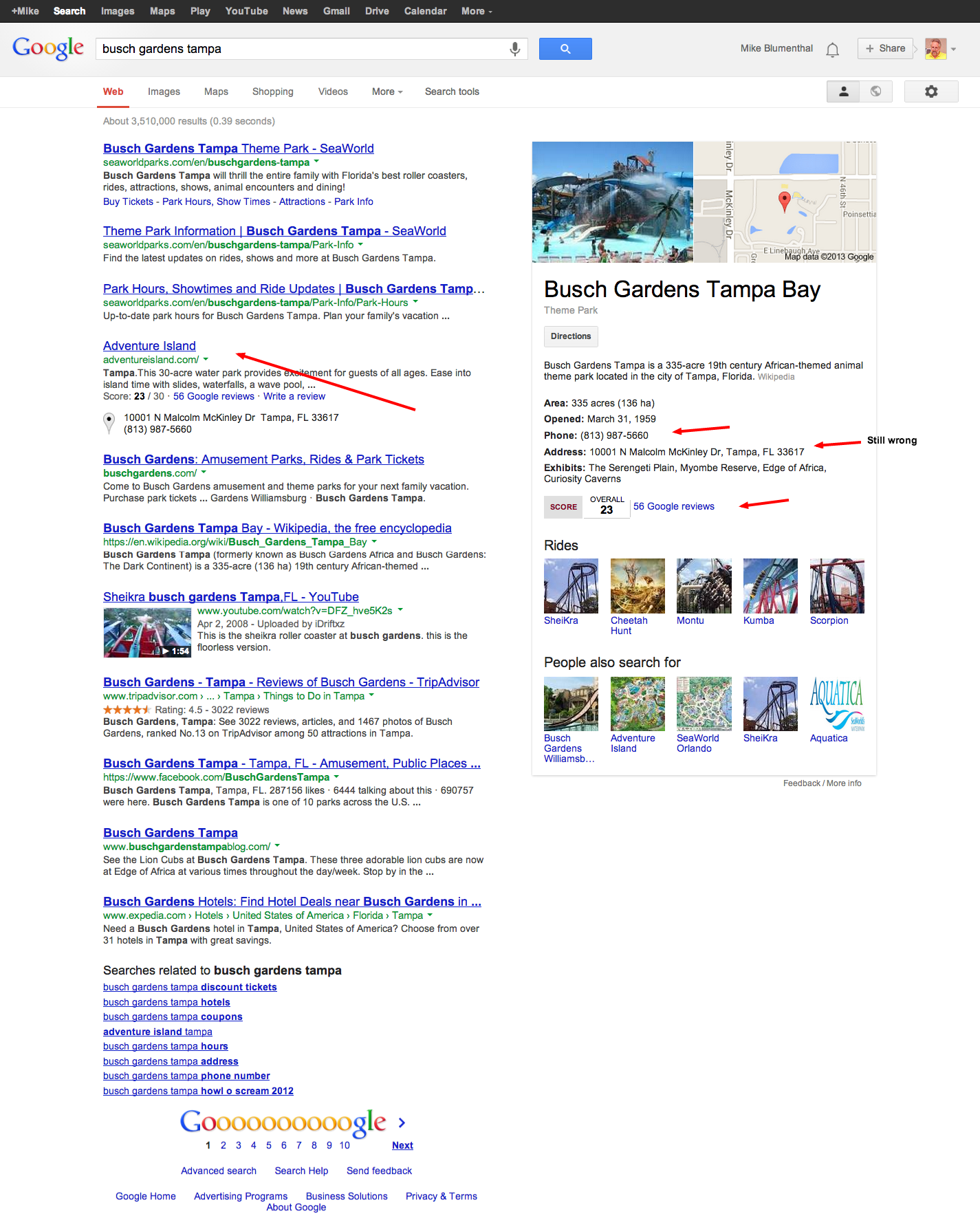The image displays a Google search results page, zoomed in, but the increased magnification does not improve readability; instead, it enlarges the interface elements. At the top, the search bar contains the query "Busch Gardens, Tampa," and the familiar Google logo with its blue, red, yellow, and green lettering is visible. Below the search bar are several search results. A prominent red arrow points to the fourth result from the top, suggesting its significance.

On the right side of the page, the Google result for "Busch Gardens, Tampa Bay" is shown. This section includes photos, a Google Maps thumbnail, and details about the location. A red arrow highlights where the phone number should be, although it’s not legible in the image. Another red arrow points to the address of Busch Gardens. Beneath these details is a blue hyperlink, also pointed out by a red arrow, but the text is unreadable due to the zoom level.

Further down, the section titled "Rides" features five thumbnail images. Below that, another section titled "People also searched for" displays five additional thumbnail images.